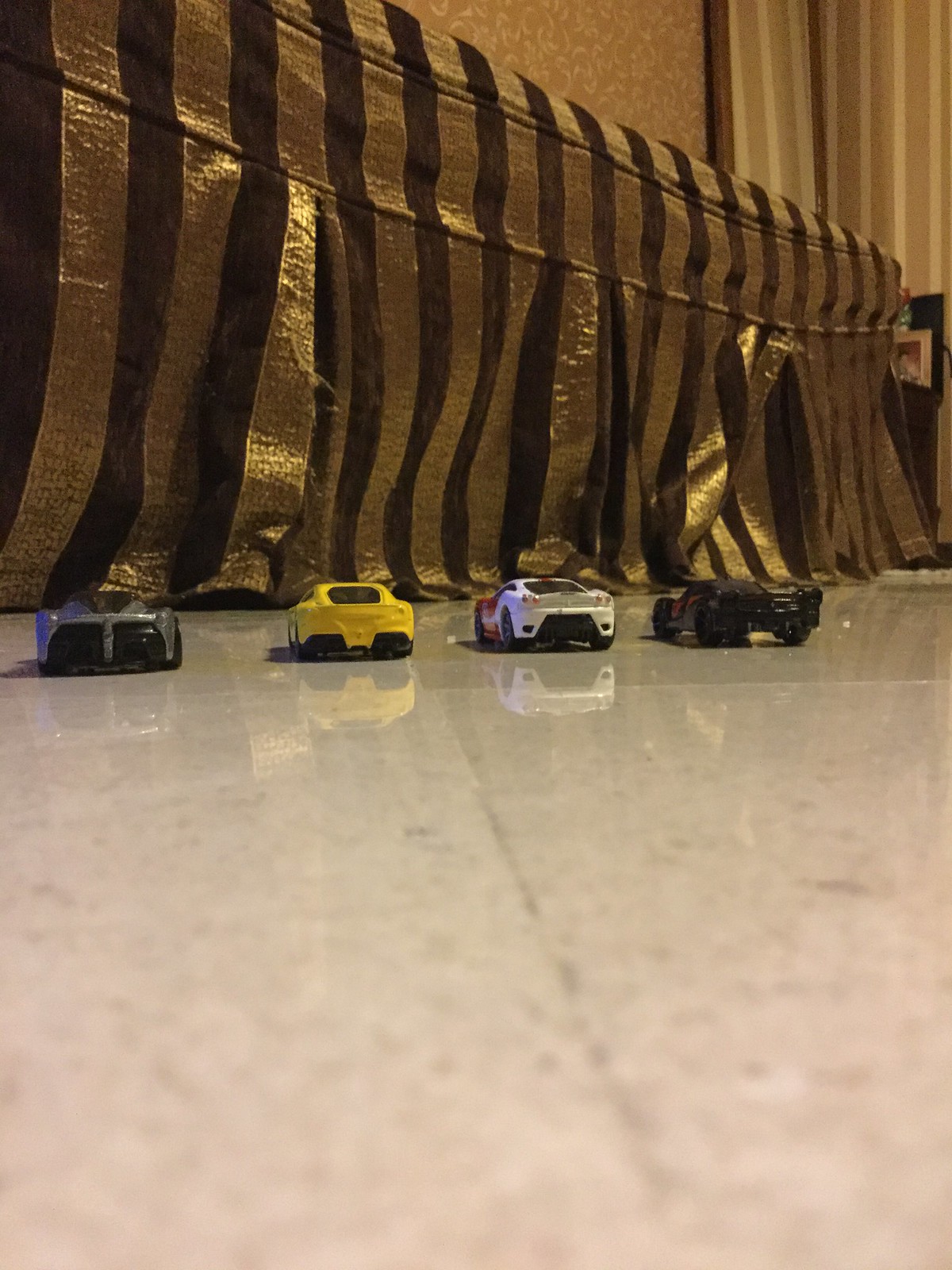The image is a color photograph taken from floor level, likely with the camera resting on a highly reflective, glossy surface that appears light pinkish-beige. In the background, there are four toy sports cars or possibly remote control cars, seen from the back. These cars are lined up side by side, from left to right, and display the following colors: gray, yellow, red and white (with white at the back and red at the front), and predominantly black. The low resolution of the image obscures finer details on the cars. In front of these cars is a piece of furniture, possibly a couch or bed, adorned with vertically striped fabric in gold and dark brown, featuring a fringed edge. The room has light-colored walls with a subtle pinkish-beige and white theme, complementing the overall gold-beige ambiance. The reflective floor surface is so polished that it mirrors the cars above it, adding to the image's intricate detailing.